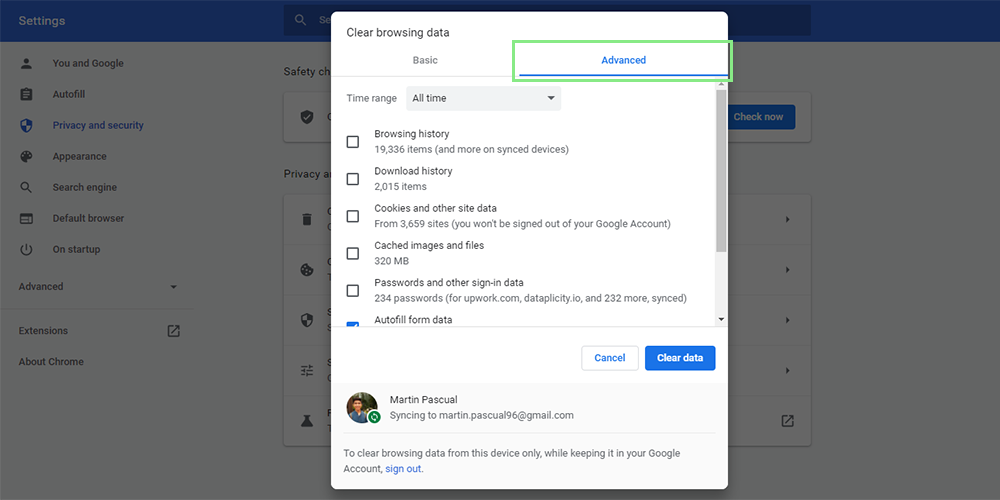The image captures a computer screen displaying the settings menu of a web browser, with a focused pop-up window titled "Clear browsing data." The settings menu in the background, located on the left side of the screen, lists several categories: "You and Google," "Auto-fill," "Privacy and security," "Appearance," "Search engine," "Default browser," and "On startup." The "Settings" header is highlighted in white text within a blue rectangular box that stretches horizontally across the screen.

In the foreground, the prominent pop-up window presents options for clearing browsing data. It offers two tabs: "Basic" on the left and "Advanced" on the right, with "Advanced" highlighted in a white box with green trimming. Below these tabs, a dropdown menu labeled "Time range" is set to "All time." The window features five selectable categories for data deletion: "Browsing history," "Download history," "Cookies and other site data," "Cached images and files," and "Passwords and other sign-in data."

At the bottom of the pop-up, there are two action buttons: "Cancel" and "Clear data," with "Clear data" emphasized in blue. Additionally, the profile information of the user, Martin Pasquale, is displayed in the lower-left corner. His avatar is shown alongside the text indicating that syncing is active under martin.pasquale96@gmail.com.